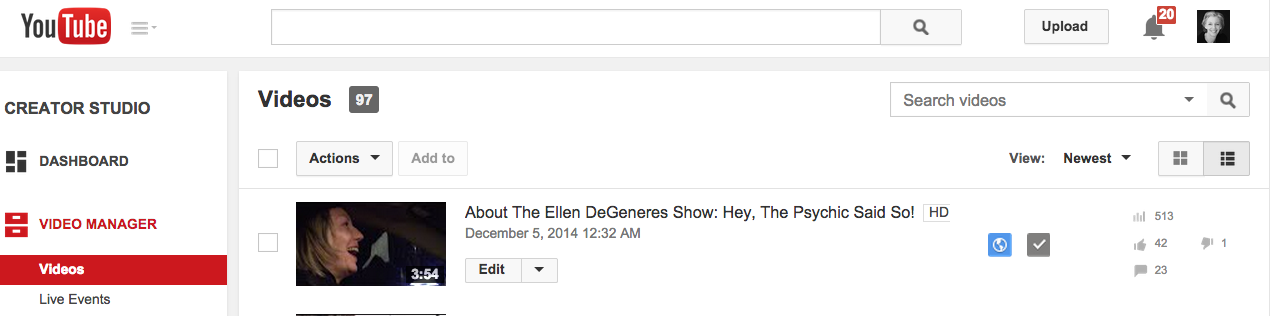This cropped image showcases the YouTube Creator Studio Dashboard in light mode. The background is white, featuring YouTube's signature red accents for highlights and selected menu items. In the upper left corner, the YouTube logo is prominently displayed next to a hamburger menu icon (three bars with an arrow) that expands for more options when clicked. An empty search bar with a magnifying glass icon sits nearby, followed by an upload button and a notification bell icon, which shows a red notification pip with the number 20. An avatar, slightly pixelated but appearing to be a black-and-white image of a woman looking towards the viewer, is located to the far right.

On the left side of the dashboard, the navigation menu displays "Creator Studio Dashboard" at the top, with "Video Manager" highlighted in red. Submenus under Video Manager include "Videos" and "Live Events," with "Videos" currently selected, indicated by a red box around it. To the right, the word "Videos" accompanied by the number 97 signifies the total video count. Below, a dropdown menu with a checkmark for bulk actions appears, as well as an individual checkmark for each video.

A recognizable video thumbnail, depicting a woman facing forward but in profile view, is visible along with the video's duration of 3:54. Part of another thumbnail can be seen below, though only a few pixels are visible. The titled video “About the Ellen DeGeneres Show. Hey, the psychic said so.” stands out in this overview of the dashboard.